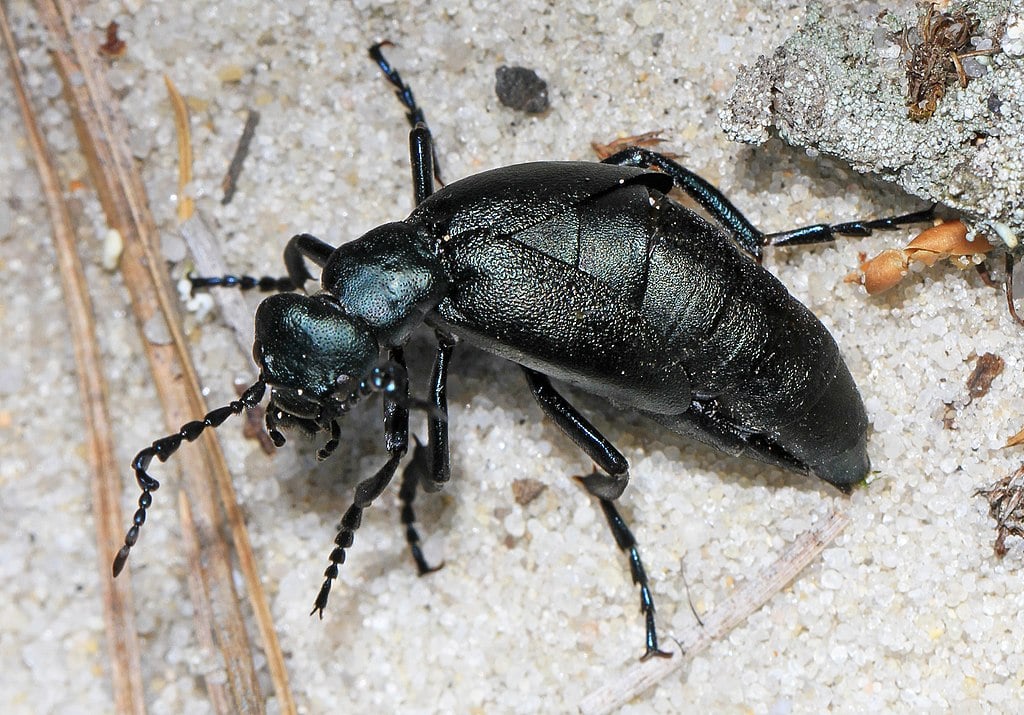The image is a detailed, close-up, color photograph of a black insect, possibly a type of ant or roach, positioned in landscape orientation. Illuminated by white light, the insect's shiny, textured exoskeleton reveals a dark green coloration with hints of iridescent green and blue, especially noticeable on its rounded head and elongated body. It has a small, round head equipped with claw-like mandibles and antennae, followed by a similarly sized upper body or thorax. The insect's body tapers into a larger, more prominent tail end or stinger area. Six segmented legs are visible extending from its sides, and there are indications it might have wings, although they are not clearly defined. The insect is depicted walking on a fine, sandy surface composed of light beige sand or tiny white rocks, interspersed with sticks and fragments of vegetation. The prominent stick on the left side of the image vertically accentuates the scene, along with additional twigs and scattered grass, adding to the naturalistic setting. The insect faces to the left and its body is slightly arched, enhancing the dynamic realism of the photograph.